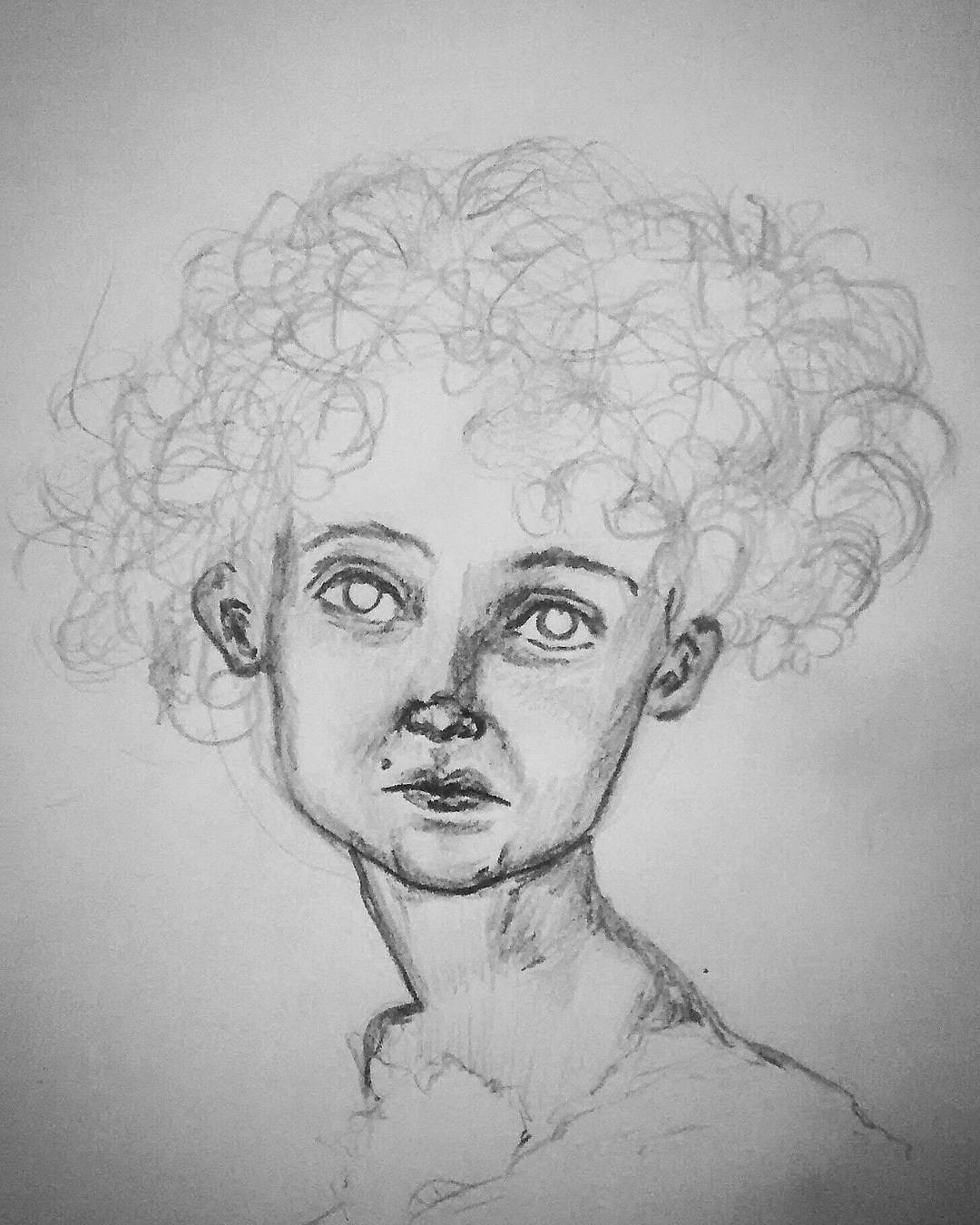This is a detailed black and white pencil drawing on an off-white, slightly grayish piece of paper. The paper appears flat and uniform, although the bottom corners are darker due to shadowing in the photograph of the drawing. The focus of the drawing is a child or a young woman, depicted from just below the neck upwards, with a slightly turned head that faces mostly forward.

The individual has a thin face with well-defined features, including a beauty mark between the nose and downturned mouth. She has large, light-colored, hollow-looking eyes that appear to follow the viewer, and well-defined eyebrows. Her nose is nicely rendered and includes visible nostrils, while her lips are realistically shaped.

One of the most striking aspects is her extremely curly, light-colored hair that occupies almost the entire width of the drawing, though it seems somewhat sparse and not densely filled in. Her ears are small and slightly protruding. The artist has also depicted a long, elegant neck and a portion of her shoulder, demonstrating considerable skill in capturing the anatomy.

The overall composition reflects a nuanced attention to detail and a profound sense of realism in the artist's depiction of the subject's proportions and facial expressions.